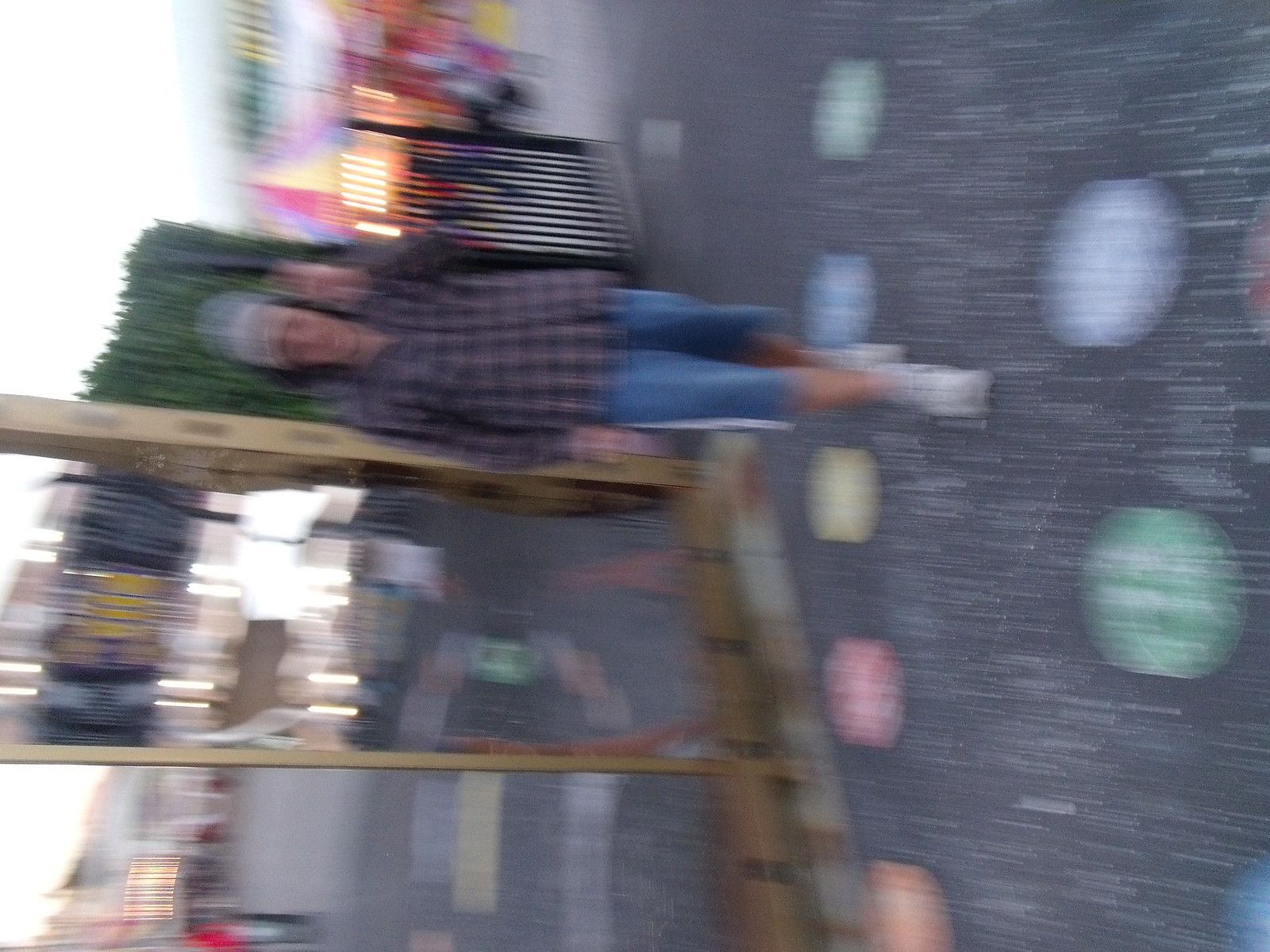In this slightly tilted and blurry image, a Caucasian individual is seen wearing a button-down plaid shirt with long sleeves, paired with blue jean shorts. On their feet are white tennis shoes. The ground beneath them is black-topped and adorned with various colored circular patterns. In the background, a wooden post and a black gate are visible, along with a building painted in vibrant shades of pink, purple, and light blue. Strings of lights add a festive ambiance to the scene.